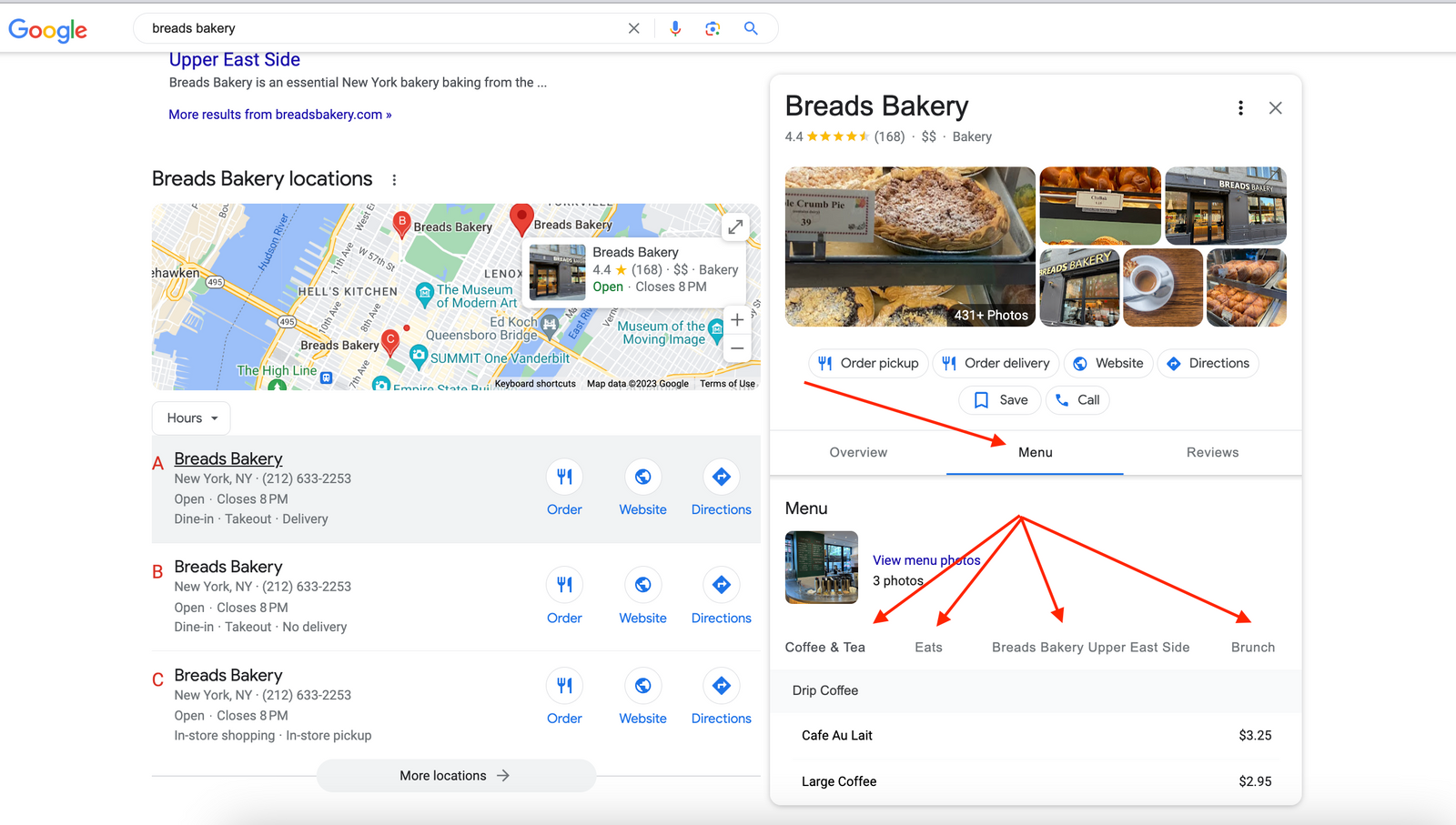The screenshot showcases a Google search result page for "Breads Bakery." The upper left corner features the iconic Google logo, with the search query "Breads Bakery" prominently displayed at the top. In the top right section, information about Breads Bakery is visible, showing a rating of 4.4 stars out of 5 based on 168 reviews. 

The results include various images related to the bakery, such as a crumb pie, several types of bread, and what appears to be a chaou, although the exact nature of this item is unclear. The pictures emphasize both the products and different views of the bakery's physical location, with signs reading "Breads Bakery."

Directly below the primary search results, there are annotations with red arrows pointing towards different categories such as "Menu," "Coffee and Tea," "Eats," "Breads Bakery Upper East Side," and "Brunch." Specific menu items listed include "Drip Coffee," priced at $2.95, "Cafe Latte" at $3.25, and "Large Coffee" at $2.95.

Further down, the screenshot suggests that there are three Breads Bakery locations in close proximity, arranged in a trailing fashion, providing various options for patrons to visit.